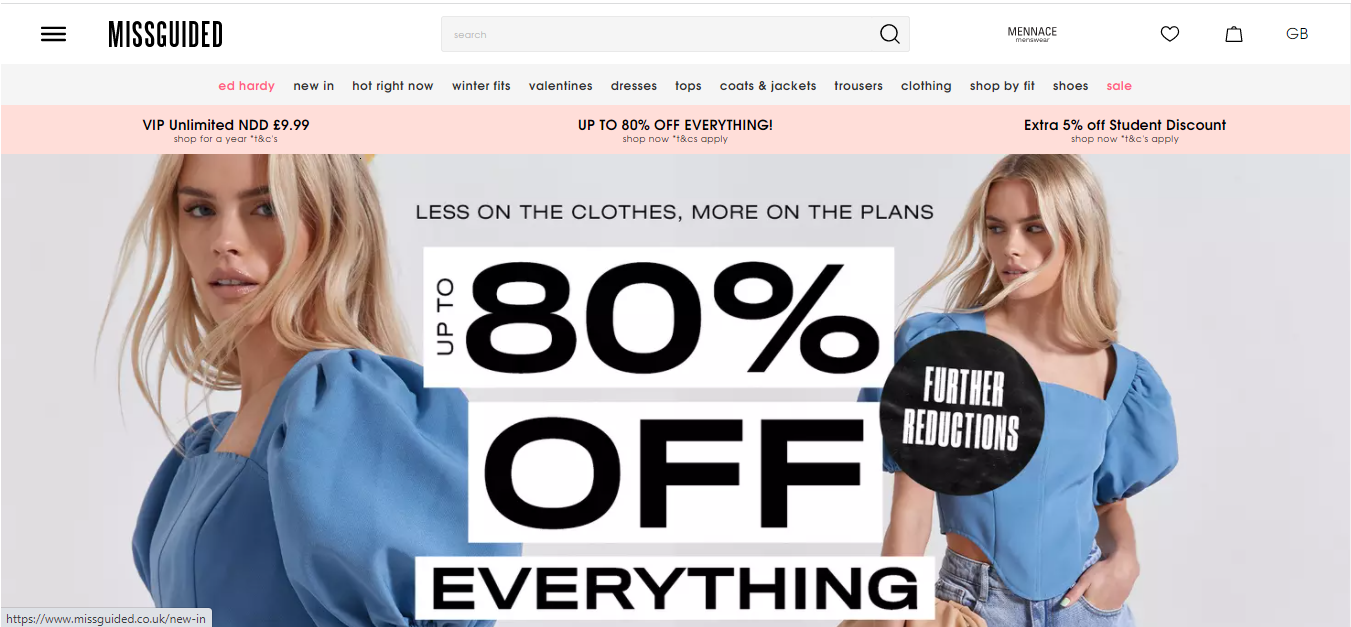Screenshot of a shopping website homepage featuring a variety of clothing options. At the top of the page, a white navigation bar displays the website's logo, "Misguided," in black on the left side, followed by a hamburger menu, a search box, and three icons on the right: a shopping bag, a heart, and an unidentifiable symbol. Below this, a series of category links are listed: "Menace" on the right (potentially a brand or collection), alongside various clothing categories such as "New In," "Hot Right Now," "Winter Fits," "Valentines," "Dresses," "Tops," "Coats & Jackets," "Trousers," "Clothing," "Shop by Fit," "Shoes," and "Sale" highlighted in red.

A pink band spans the page beneath the categories, advertising "VIP Unlimited" for £9.99 per year, which offers benefits such as next day delivery. Further promotions include "Up to 80% Off Everything" and an "Extra 5% Off Student Discount," alongside mentions of applicable terms and conditions. 

Central to the page is an image with a grey background showing a woman with long blonde hair and tan skin. On the left side, she is more zoomed in, wearing a square-neck blue top with puffed sleeves extending to her elbows, styled in a V-shaped cropped design, paired with light blue jeans or shorts. The image is overlaid with text stating, "Less on the clothes, more on the plans," highlighting the "Up to 80% Off Everything" sale. Additionally, a circular badge on the right side of the image announces "Further Reductions."